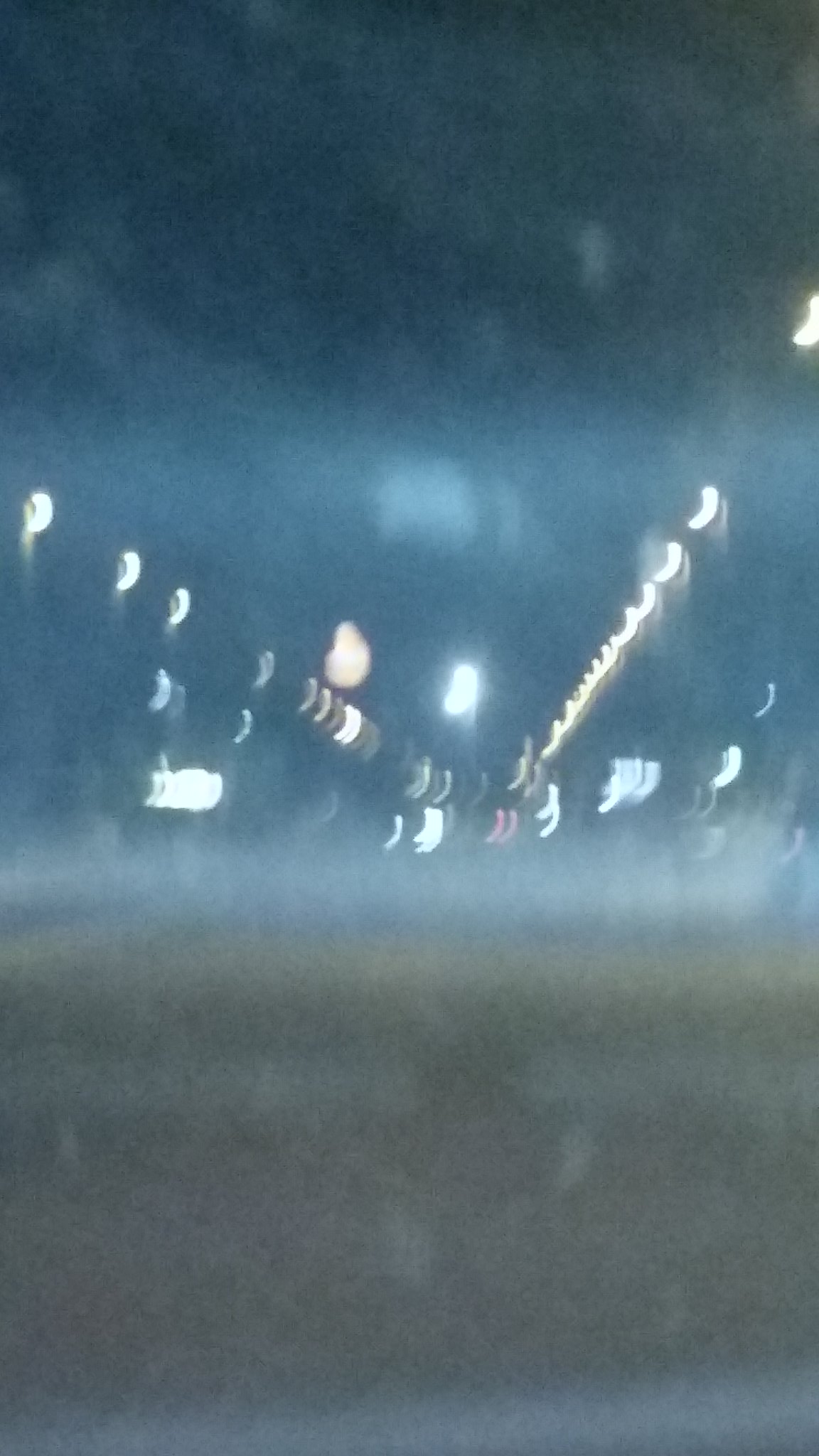The image is a very blurry and grainy photograph, likely taken from the inside of a car through a rain-spattered windshield, which distorts the overall view. The photo, possibly of a highway at nighttime, features an array of light reflections, giving it an almost halo effect. Predominant colors in the image include shades of yellow, gold, black, and white, with a few red lights in the distance likely indicative of vehicle taillights. The road itself is somewhat discernible despite the blurriness, with the glassy, dirty look from water droplets and mist contributing to the difficulty in making out clear details. The lights, both on the left and right sides and in the background, create a shiny effect, with some appearing yellow or white and possibly originating from headlights or streetlamps. At the top of the image, a bluish-gray sky is visible, adding to the image's overall rainy, nighttime ambiance.